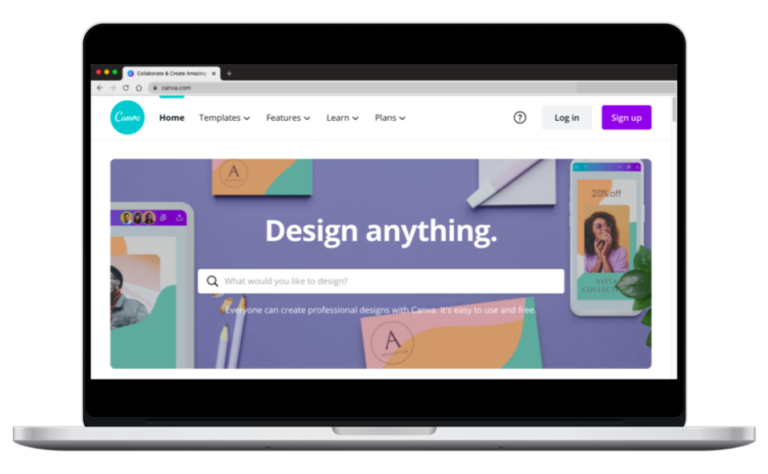Promotional Image for Canva on a MacBook:

The image is a promotional shot of a MacBook laptop, expertly edited to showcase the device in an engaging way. At the very bottom, the sleek silver base of the laptop is visible. Above it, the screen is folded open, presenting the Canva website interface in fine detail. Though the printing is small, the user interface can be discerned, featuring main menu categories such as Home, Templates, Features, Learn, Plans, along with icons for Help (question mark), Login, and Sign Up.

The central portion of the screen is vibrant with intertwined graphics in shades of purple, orange, mint, teal, and green, and features a bold white text headline, "Design Anything." Just beneath this, a clickable search bar invites users with the prompt, "What would you like to design?" Below the search functionality, a reassuring message reads, "Everyone can create professional designs with Canva. It's easy to use and free."

The familiar layout and design elements strongly suggest the laptop model is a MacBook, mirroring the setup on the user's own computer, further underlining the intuitive and user-friendly experience Canva aims to provide.